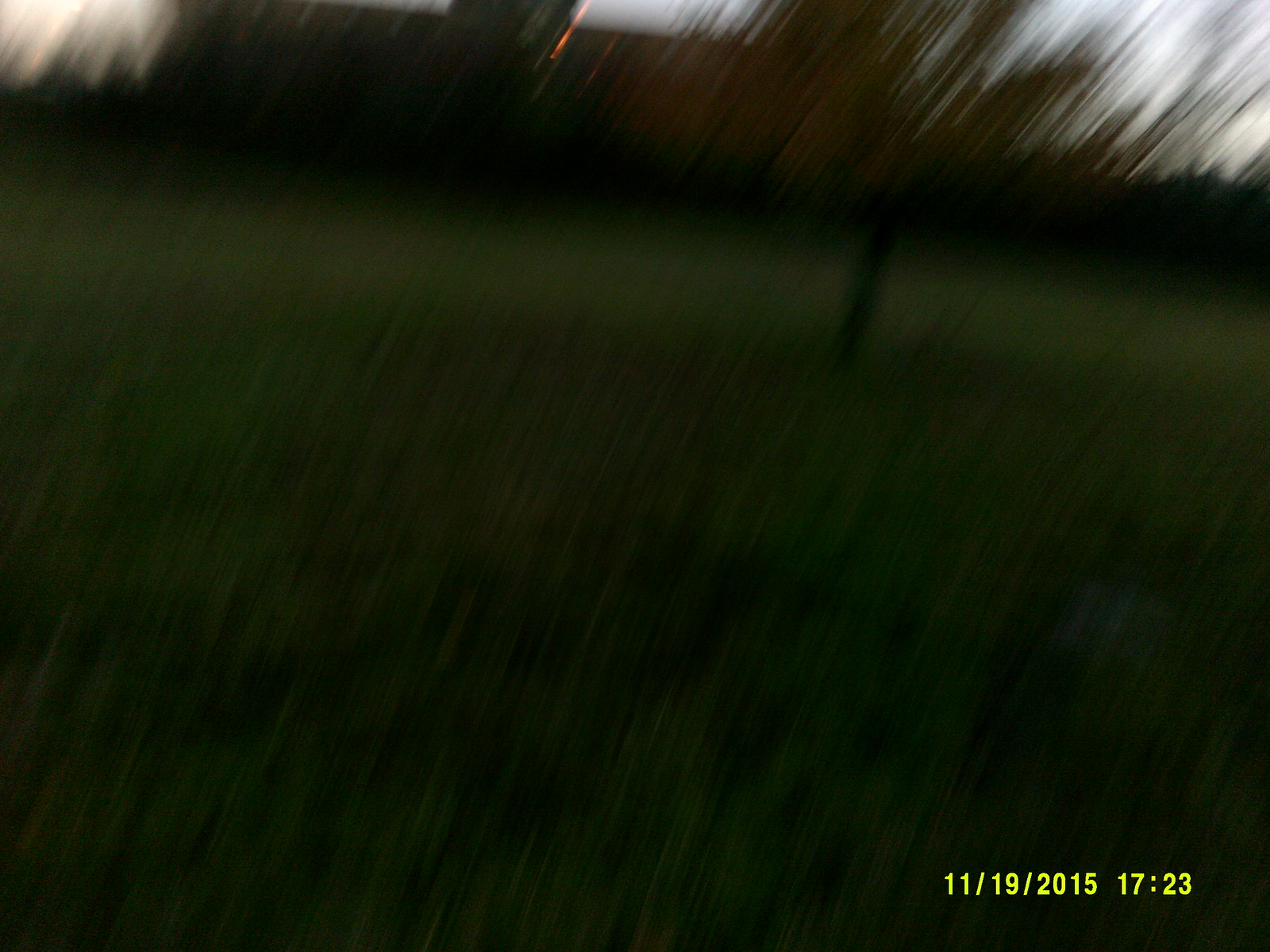This photograph, taken outdoors on November 19, 2015, at 17:23 (5:23 PM), is a highly blurred image that seems captured while the camera was in motion. Dominated primarily by tall, slightly darker green grass at the bottom and lighter, longer grass extending higher up, the entire scene is characterized by streaky, line-like distortions going from the bottom left to the top right, giving an impression of chaotic, child-like scribbling. In the backdrop, there is an indistinct silhouette of what appears to be a building, potentially made of reddish brick, along with another darker silhouette which might be a tree. Among these indiscernible features, there is a faint orange flicker, possibly a distant light. This entire scene, tilted to the right, is further contextualized by the yellow timestamp at the bottom right corner of the image reading "11/19/2015 17:23."